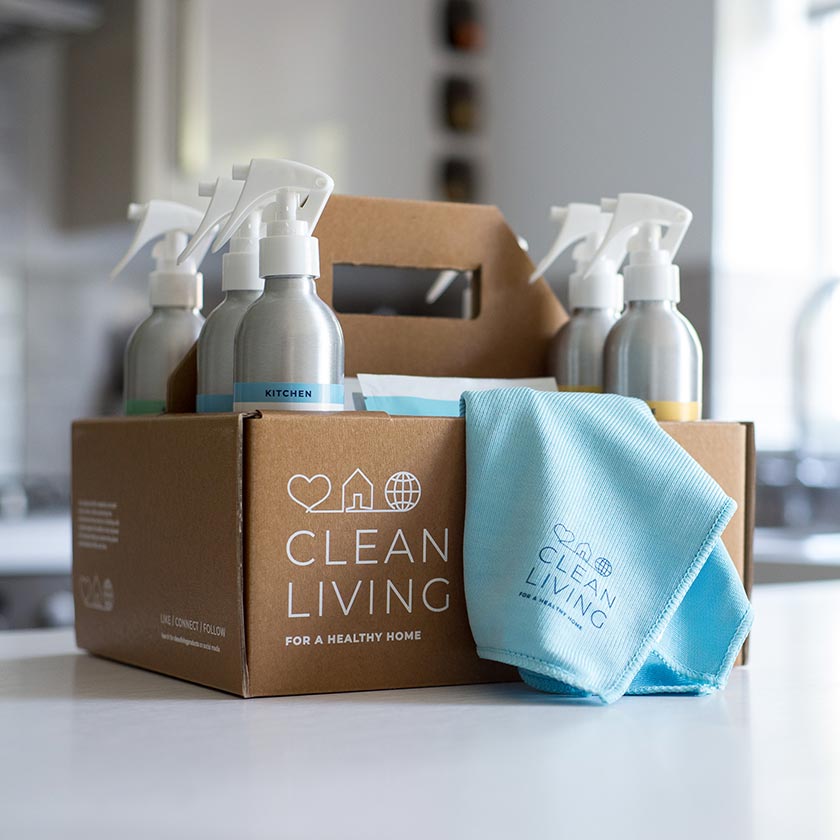The indoor photograph, taken during the daytime, captures a neatly organized brown cardboard caddy positioned slightly to the right on a light gray countertop. The caddy functions as both a container and a carrying case, featuring a central handle. Prominently displayed on the caddy is white text that reads “Clean Living for a Healthy Home,” accompanied by icons of a heart, house, and globe. Inside the caddy, there are six sleek spray bottles with white caps, designed in a brushed metal finish that adds a touch of elegance to the cleaning products. Draped over the right-hand side of the caddy is a light blue microfiber cloth, also branded with the "Clean Living for a Healthy Home" text. The blurred background, likely a kitchen as indicated by a faintly visible faucet, emphasizes the caddy and its contents, suggesting a focus on cleanliness and home care. The image, square in shape and approximately 5x5 inches, subtly hints at a possible advertisement for this line of cleaning products.